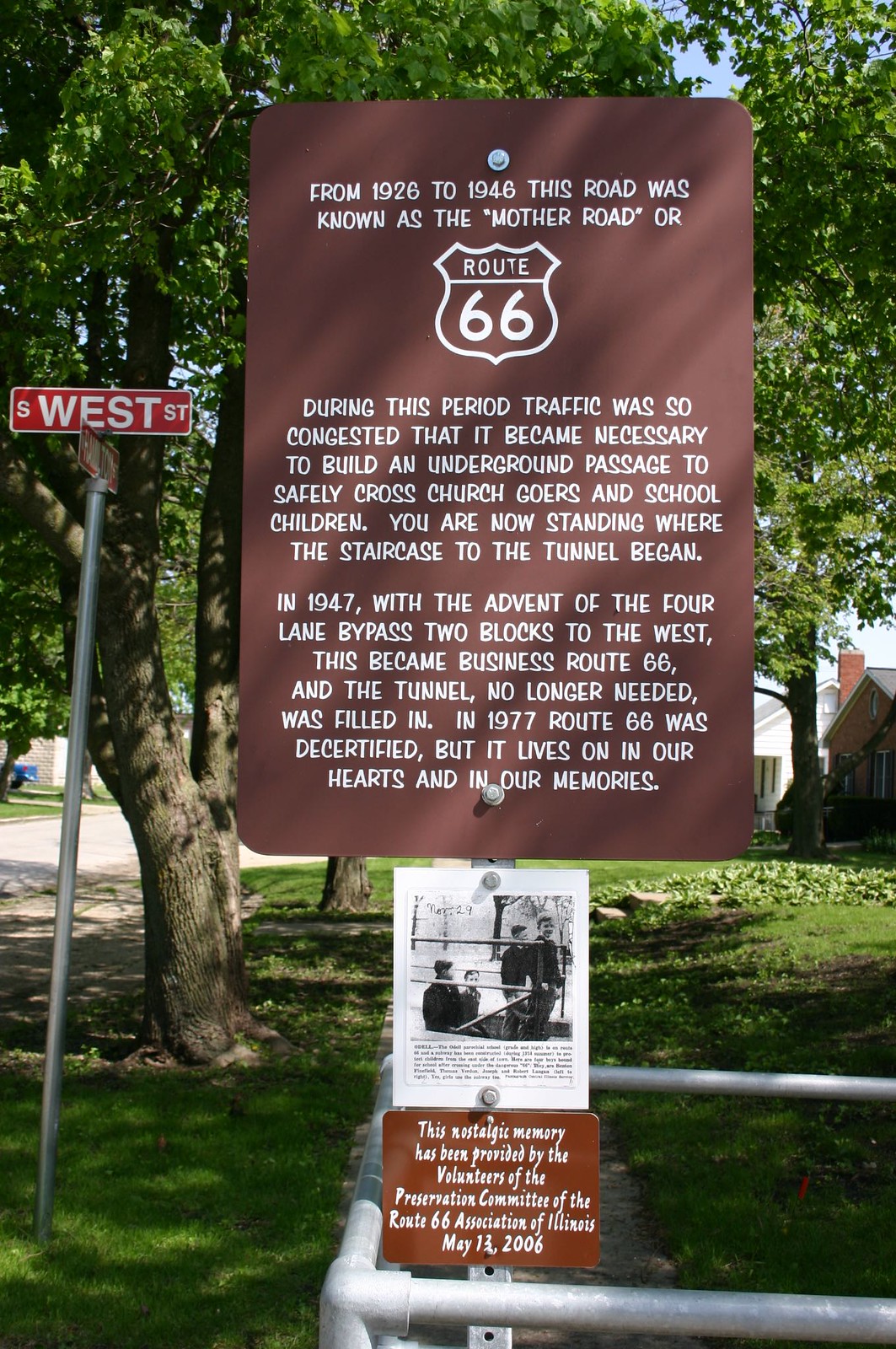This photograph captures a historic marker for Route 66, taken outdoors in a park setting, with lush green trees in the background. The image is in portrait mode, making it taller than it is wide. Central to the photo is a brown sign with white lettering, detailing the rich history of this celebrated road. It reads:

"From 1926 to 1946, this road was known as the Mother Road or Route 66. During this period, traffic was so congested that it became necessary to build an underground passage to safely cross churchgoers and schoolchildren. You are now standing where the staircase to the tunnel began. In 1947, with the advent of the four-lane bypass two blocks to the west, this became Business Route 66 and the tunnel, no longer needed, was filled in. In 1977, Route 66 was decertified, but it lives on in our hearts and in our memories."

Beneath the historical description is a black-and-white photograph of four men, illustrating the past significance of this location. Below the photograph, another sign credits the Preservation Committee of the Route 66 Association of Illinois, dated May 13th, 2006, for preserving this nostalgic memory. To the left, the street sign for West Street in red with white lettering on a gray metal post adds to the historical ambiance of the scene.